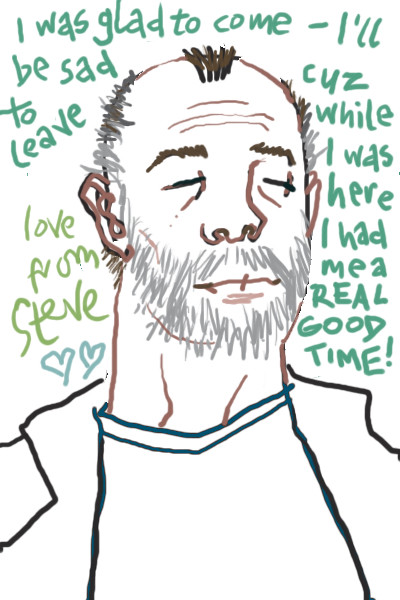This vertically-aligned rectangular image features a hand-drawn caricature of a man against a white background. The drawing, created with various colored markers, showcases the man’s mostly bald head, featuring a few vertical spikes of brown hair on top and some squiggly lines of brown and gray on the sides. His bushy eyebrows are colored brown, complemented by closed, slitted eyes filled in black and brown. The man's prominent nose is outlined in brown, while his ears and neck follow the same brown outline. He sports a scruffy gray beard and mustache.

He is depicted wearing a t-shirt and a jacket, with his shoulders outlined in black. Surrounding the man’s head is a handwritten message in green marker. At the top, it reads, "I was glad to come. I'll be sad to leave." Down the right side, the message continues, "cuz while I was here I had me a real good time!" In a different shade of green on the left side near the neck area, the note concludes with "Love from Steve," accompanied by two blue hearts.